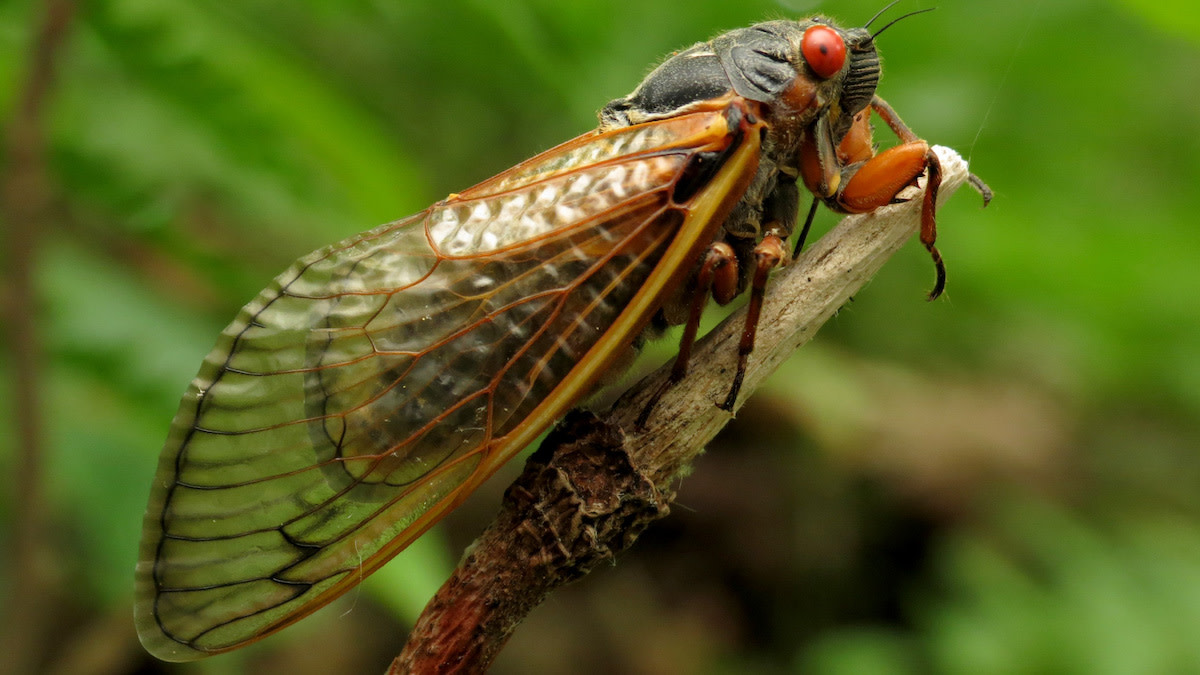This close-up, detailed photograph captures a large horsefly-like insect perched on the end of a branch, which has a bit of white at its tip. The insect features prominent, bulging red eyes with black centers and slightly hairy, brown legs. Its striking wings are transparent, revealing a mixture of gold and brown hues towards the top, transitioning to green near the edges, with orange outlines. The insect's body is elongated with brown tones. The background showcases an out-of-focus array of green foliage, including leaves, bushes, and blurred trees that enhance the focus on the insect's detailed anatomy. The insect, possibly a type of hopper, has a notable wingspan and six legs, with two tentacle-like appendages.